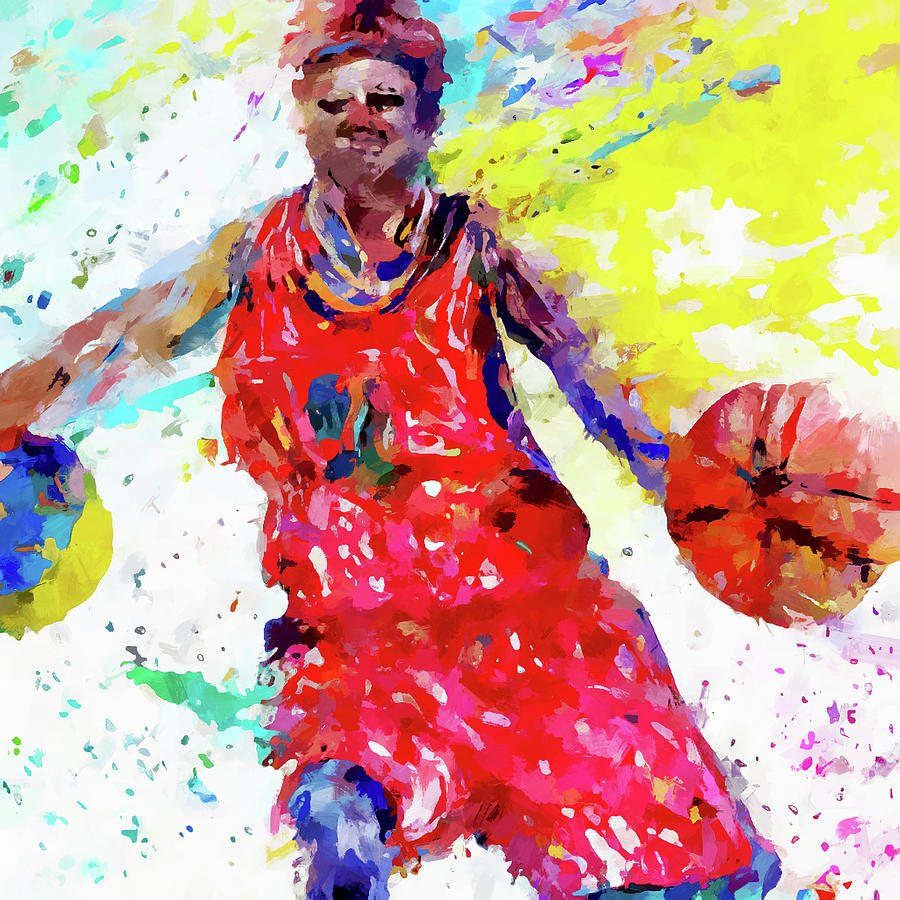This artwork is an original, vibrant, and modern acrylic painting depicting a basketball player in the center against a white background. The player, a person of color, is wearing a bright red jersey and red shorts. He holds an orange basketball in his left hand, which features highlights of yellow and black. His right hand, semi-hidden and possibly holding another object appearing like a multi-colored ball, features shades of yellow, aqua blue, and darker blue. The player has a distinctive headband and a tuft of red and black hair, with an indistinct facial expression that hints at a mustache and barely visible black hair. His uniform displays an abstract symbol that may represent his team. Surrounding this central figure are splashes and splotches of vibrant colors including yellow, aqua, pink, white, peach, turquoise, blue, and speckles of purple, creating a dynamic and colorful background. The dimensions of the painting are approximately 8 1⁄2 inches wide by 9 1⁄2 inches long, giving it an almost square shape. The overall style is modern and slightly abstract, with no text included in the image.